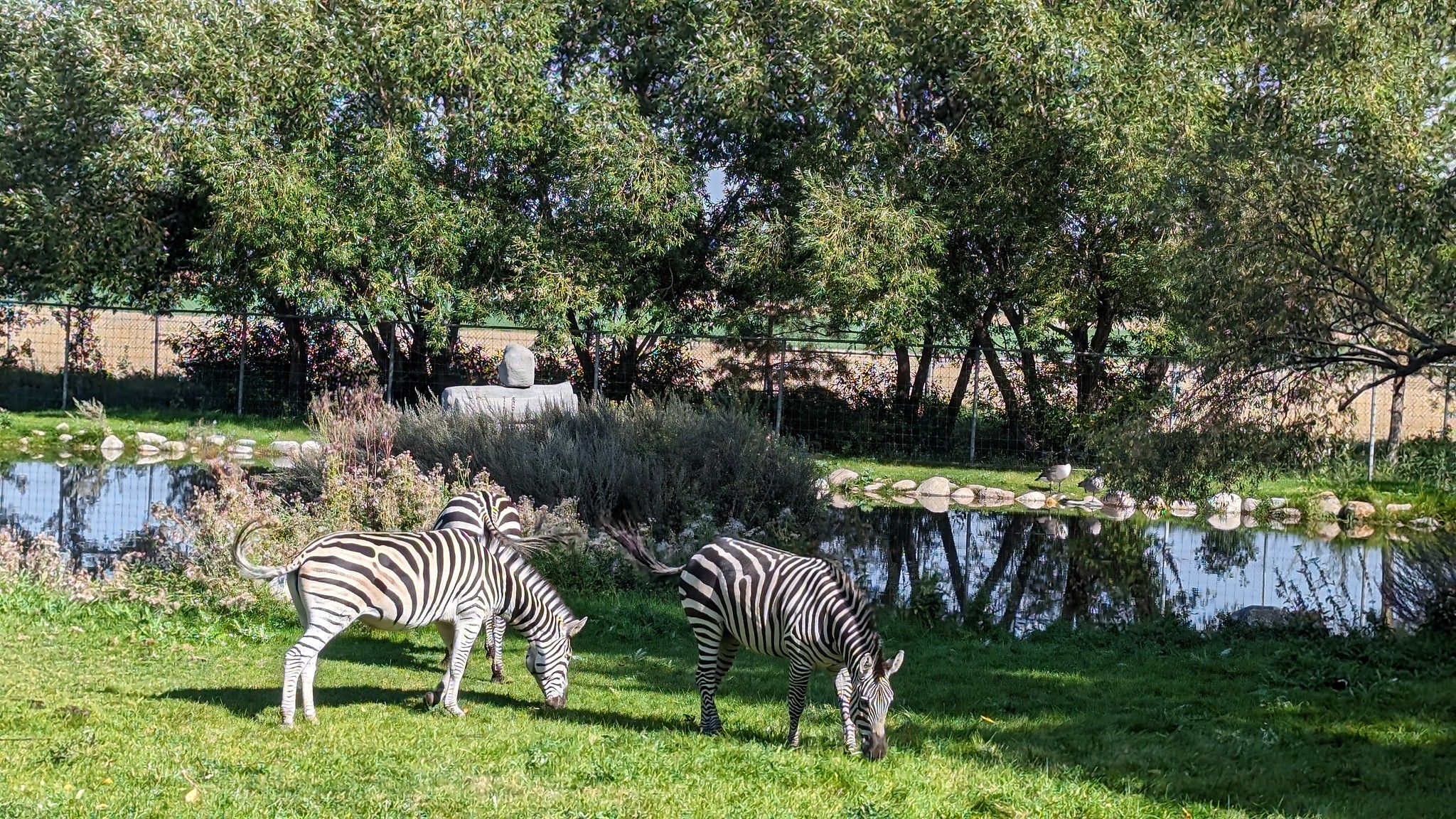In this detailed image, three adult zebras with distinctive black and white stripes are grazing on lush green grass in a seemingly man-made enclosure. The two zebras in the foreground are facing to the right with their heads down, while the third zebra is partially obscured behind them, showing only its rear end and facing away from the camera. The scene is set against a tranquil, glassy pond that reflects the surrounding landscape, indicating very little to no current. The pond is bordered by cobblestones, adding to the artificial appearance, and there is a stone statue or monument partially visible on the opposite side.

The background boasts a dense line of mature, leafy deciduous trees. Somewhere on the right side of the image, a couple of birds, possibly ducks, are seen near the cobblestones. The enclosure is demarcated by a combination of a wire fence and a more substantial pale wooden fence behind the pond. Beyond the fence, there is a hint of another open, green area. A large bush is positioned near the zebras, and the sky features small peek-throughs of blue. The entire scene is bathed in natural daylight, emphasizing a serene and picturesque setting, likely in a wildlife park or a similar controlled environment.